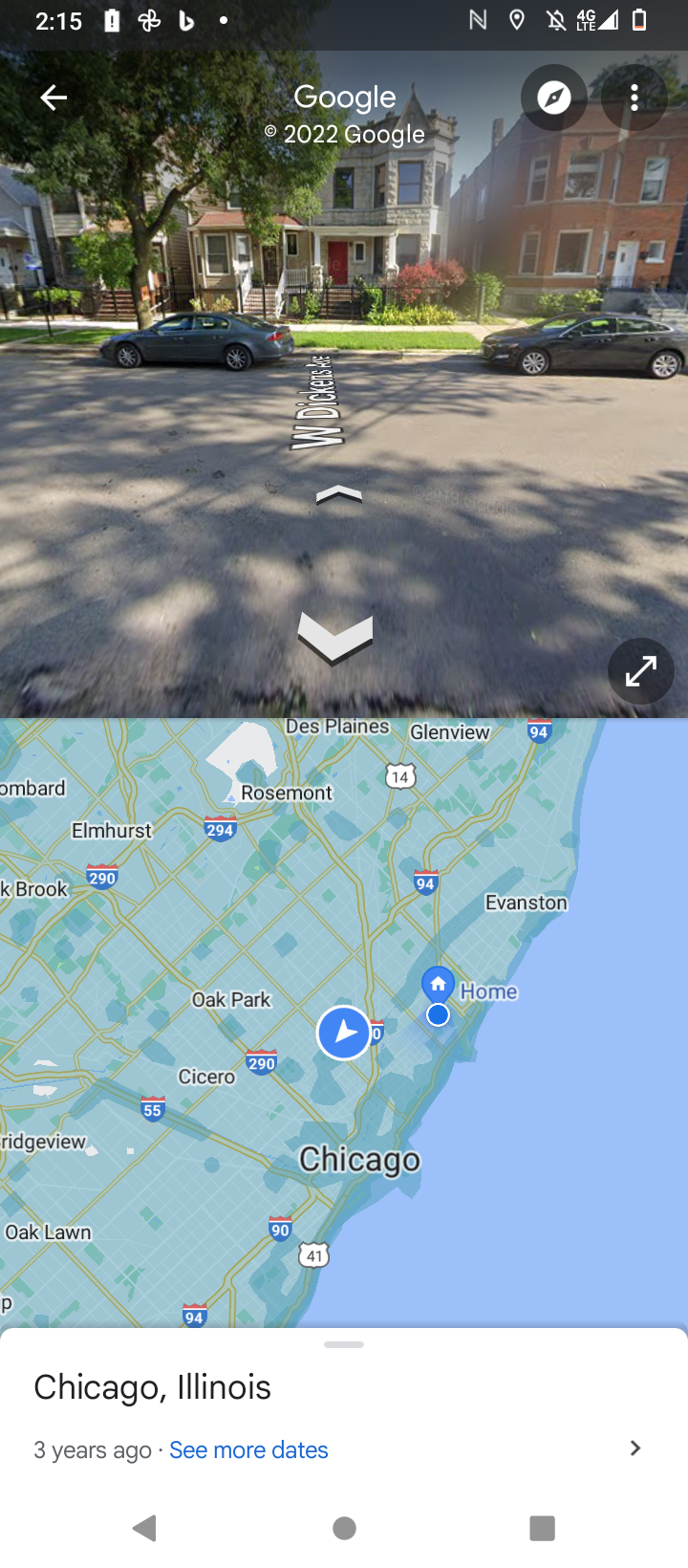This is a screenshot from a mobile phone displaying Google Maps, with a clear view of the phone's user interface icons. At the top left, the clock reads 2:15, alongside various app icons. On the right, icons indicate GPS, 4G LTE connectivity, signal strength, and remaining battery life. The screen is divided; the top half features a Google Street View rendering of a residential area on West Dickens Avenue in Chicago, Illinois, showing two cars parked in front of a brownstone-style house with a black fence and well-landscaped garden. Surrounding are other large homes, suggesting a pleasant, residential neighborhood. The bottom half of the screen presents a satellite or aerial view map, pinpointing the location within Chicago. The map data appears to be from 2022, indicating it may not be the most current. Bottom screen controls are visible, further indicating interactive map features.